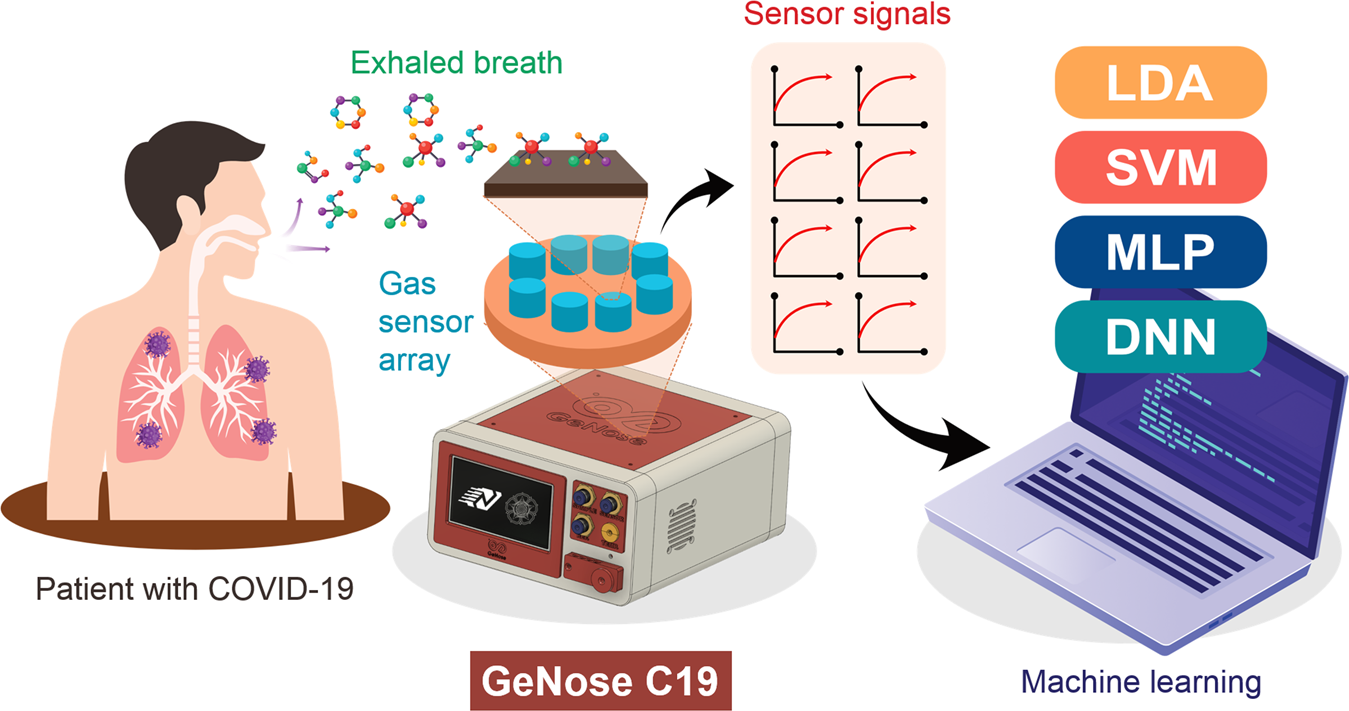This detailed illustration, reminiscent of an educational poster or textbook page, provides a comprehensive visual explanation of a COVID-19 testing mechanism involving a patient and machine learning processes. On the left, a cartoon-style cross-section image of a man is shown, identified as a "patient with COVID-19," with a clear depiction of his respiratory system including the lungs, sinus, and bronchial areas. The lungs are detailed with purple COVID-19 particles. The man is exhaling tiny molecules, labeled as "exhaled breath," which lead to a "gas sensor array" situated in the middle of the image.

This sensor array resembles a red and white box, akin to a microwave, with various knobs and a brown plate topped with blue cylinders. Above these cylinders, an orange triangle interacts with the exhaled molecules. Below this device, text reads "GE NOSE C-19," likely indicating the name of the testing apparatus, potentially pronounced as "G knows COVID-19."

To the right of the gas sensor array, the image transitions to the data interpretation stage, depicting several small parabola-shaped charts labeled "sensor signals." These charts connect via arrows to a purple laptop signifying the "machine learning" component. Above the laptop, in separate labeled boxes, are different machine learning techniques: LDA (Linear Discriminant Analysis), SVM (Support Vector Machine), MLP (Multi-Layer Perceptron), and DNN (Deep Neural Network).

The entire scene is vibrantly colored, designed to convey the sequential process from detecting exhaled breath through a sensor array to analyzing the data using machine learning on a laptop, effectively visualizing how COVID-19 patient data is interpreted.